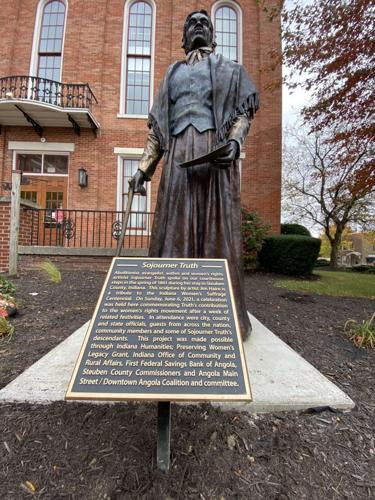This image features an iron statue of Sojourner Truth situated outdoors in front of a red brick building with multiple windows, balconies, and a lower level encircled by a railing. The statue depicts Sojourner Truth dressed in a long black dress paired with a blue vest, topped with a black shawl, and accented with a scarf around her neck. She holds a piece of paper and a cane in her hand. Surrounding the platform on which the statue stands, there are green shrubs, grass, and a red-leaved tree. In front of the statue, there's a plaque with gold lettering on a black background, which somewhat legibly notes that the project was made possible through Indiana Humanities Preserving Women's Legacy Grant, Indiana Office of Community and Rural Affairs, First Federal Savings Bank of Angola, Steuben County Commissioners, and Angola Main Street.